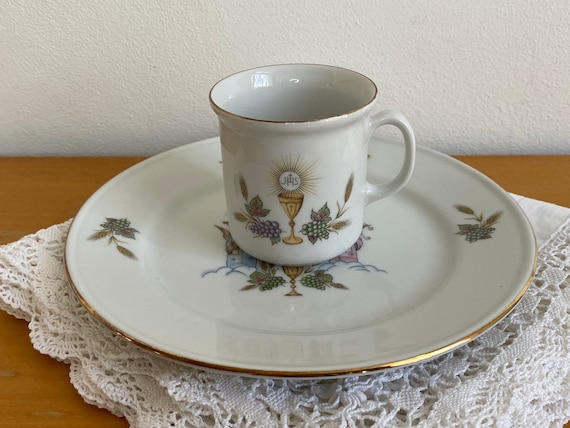The image features a white teacup with a classic mug shape, adorned with gold accents on its rim, and a matching white saucer. Both the teacup and the saucer boast a detailed design, primarily showcasing a gold chalice marked with a cross, surrounded by grape clusters, grape leaves, and wheat stems forming a U-shape around the chalice. The matching plate, which repeats this intricate artwork, sits atop a neatly folded white lace doily, further accentuating its delicate appearance. All these elements rest on a polished brown wooden table, contrasting subtly with the simple white wall backdrop, ensuring the elegant display of the teacup and saucer is the focal point of the photograph.